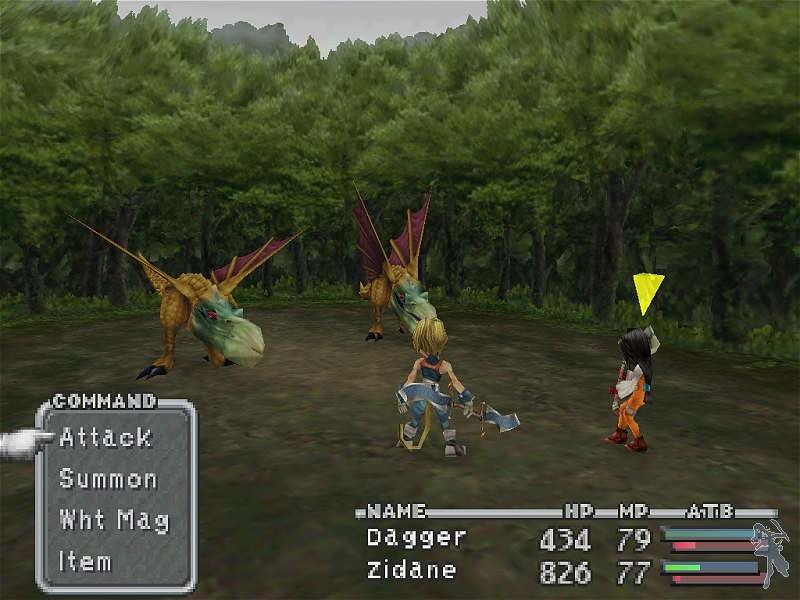The image is a detailed screenshot from the PlayStation-era game, Final Fantasy 9, featuring a battle scene set in a forest clearing. The scene's background showcases a pixelated, off-blue sky and solid green, digital-looking trees with brown trunks. The forest floor is brown, with patches of green suggesting grass. 

In the center of the screen, two human characters, Dagger and Zidane, are poised for battle against two dragon-like creatures. The dragons boast orange bodies with green heads, bright red eyes, large beaks, purple wings with yellowish markings, and black talons. Dagger, the currently selected character, has a command box at the bottom left of the screen highlighted with a white border and filled with dark gray. The command options displayed in white text are "Attack," "Summon," "Wht Mag," and "Item."

At the bottom right of the screen, the status for Dagger and Zidane is displayed, showing their names, HP, and MP values. Dagger has 434 HP and 79 MP, while Zidane has 826 HP and 77 MP. The battle is set during the daytime, adding to the clarity and detailing of the game’s vintage graphics.